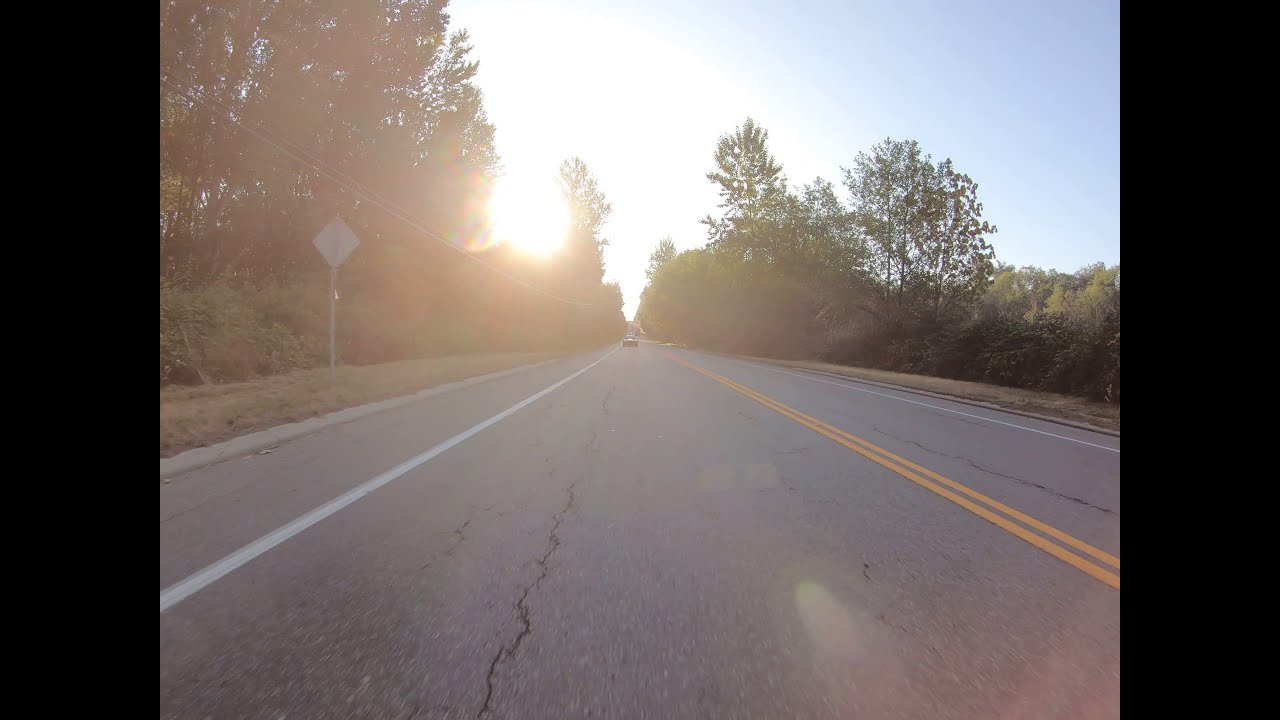The image depicts a remote, two-lane road stretching into the distance, bordered by solid white lines on the edges and a double yellow line in the center indicating different lanes of traffic. Dominating the center of the image, the road is flanked by lush, dark green trees with thin branches, largely overhanging the roadway. A single dark-colored car is visible in the distance, partially obscured by the sun's bright beams shining through the foliage at the top center of the image. The sky is mostly light blue with no clouds, adding to the serene outdoor setting, captured from the perspective of someone standing on or driving down the road. A couple of signs—including a diamond-shaped one just out of view—can be glimpsed alongside the road, and power lines stretch across the top left corner of the image. The overall scene is bathed in natural light, likely taken during the middle of the day.